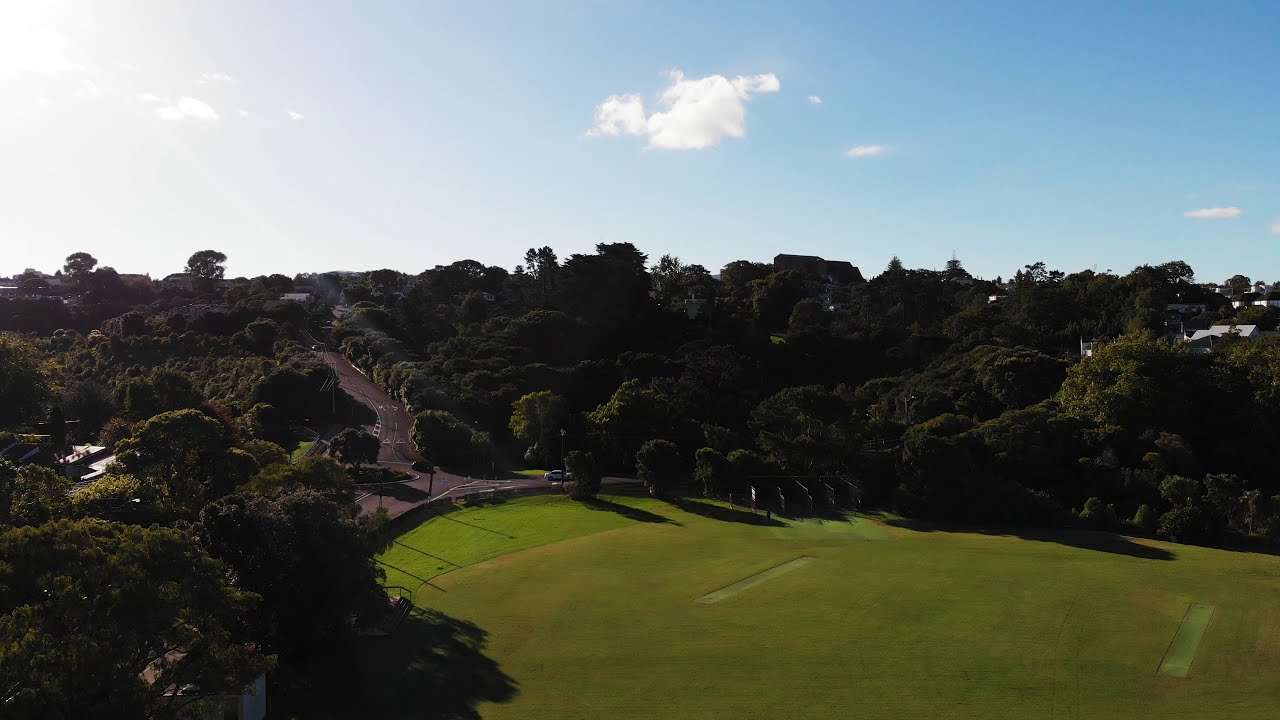The image depicts a vast, verdant landscape that appears to be a golf course or a versatile green area, potentially used for various recreational activities such as soccer. The snapshot seems to have been taken from a high vantage point, overlooking an expansive field that stretches out towards a clear, blue sky adorned with a few white, puffy clouds. It’s either early morning or dusk, as the low-hanging sun casts silhouettes of the abundant trees scattered throughout the scene.

A dense cluster of trees forms a semicircle around the central green area, their lush foliage suggesting a midsummer or late spring setting. Hidden within these trees are several rooftops, hinting at nearby houses or businesses. Two intriguing rectangular imprints are visible on the well-maintained grass, possibly indicating areas for portable goals or moveable equipment, enhancing its utility for different sports.

On the right-hand side of the image, the grass transitions to a slightly duller hue and appears freshly mown, reinforcing the golf course impression. A few flags and what might be storage areas are visible along the edge. Surrounding the green expanse, roads wind their way up gentle hills, and a solitary white car is parked in a small lot, with no other vehicles in sight. The picturesque scenery is bathed in soft sunlight, adding to the tranquil ambiance of this probably multi-use recreational space.